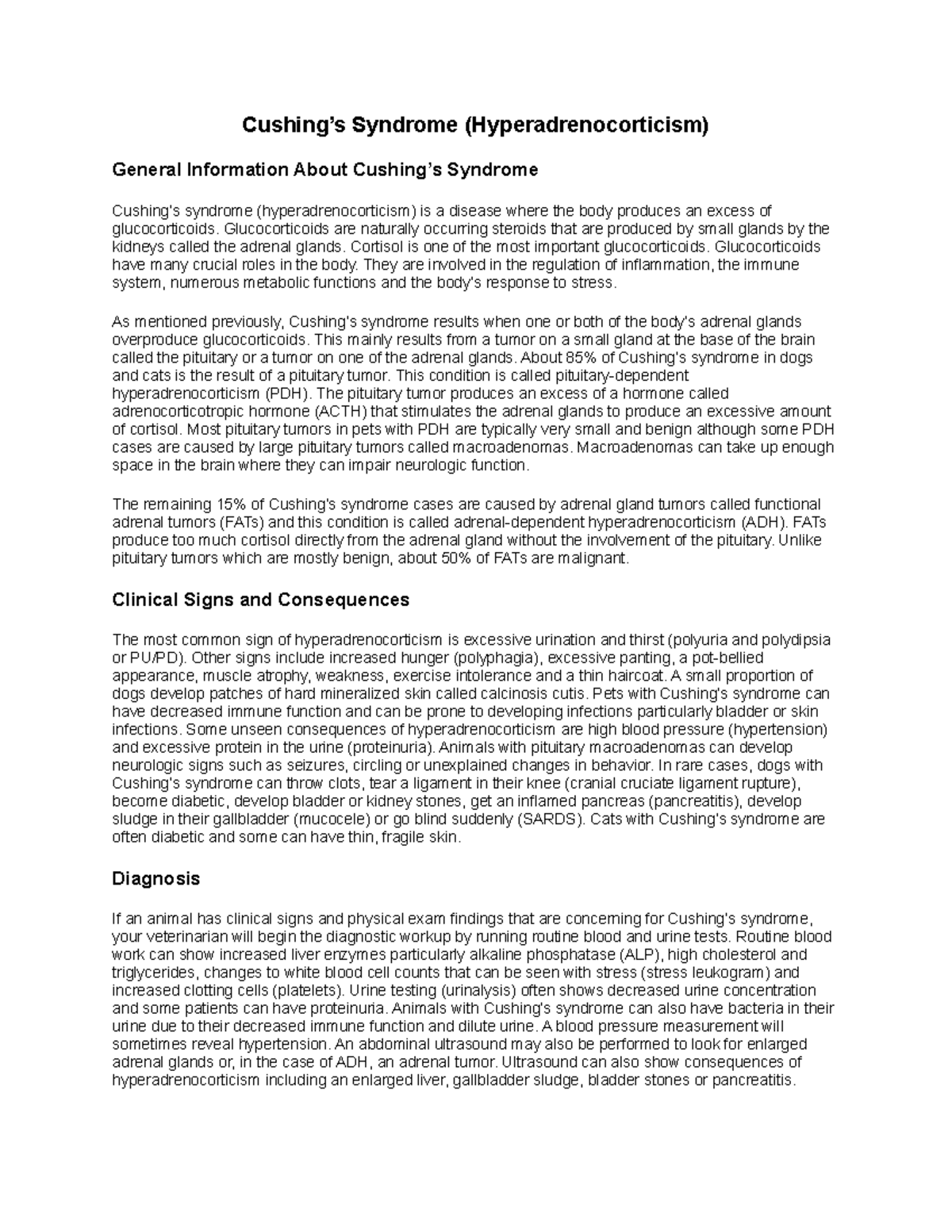#### Detailed Caption for Image:

The image showcases an article on a white background with black text, thoroughly detailing Cushing's Syndrome, also known as Hyperadenocorticism. The headline of the article reads: "Cushing's Syndrome, Hyperadenocortisism: General Information about Cushing's Syndrome."

The article provides an in-depth explanation of this disease in which the body produces an excess of glucocorticoids, naturally occurring steroid hormones produced by the adrenal glands located near the kidneys. Cortisol, a crucial glucocorticoid, plays significant roles in regulating inflammation, the immune system, metabolic functions, and the body's response to stress.

Cushing's Syndrome primarily results from either a pituitary tumor (Pituitary Dependent Hyperadenocorticism, PDH) or an adrenal gland tumor (Adrenal Dependent Hyperadenocorticism, ADH). PDH, affecting around 85% of cases in dogs and cats, stems from a small benign or, occasionally, large pituitary tumor that produces excessive adrenocorticotropic hormone (ACTH), stimulating overproduction of cortisol by the adrenal glands. On the other hand, ADH occurs when adrenal tumors directly secrete excessive cortisol, with about 50% of these tumors being malignant.

The article lists clinical signs of Hyperadenocorticism, including excessive urination and thirst (polyuria and polydipsia), increased hunger (polyphagia), muscle atrophy, weakness, thin haircoat, and sometimes mineralized skin patches (calcinosis cutis). Neurological symptoms, high blood pressure (hypertension), and excessive protein in the urine (proteinuria) can also occur. Severe cases may lead to complications such as diabetes, ligament tears, pancreatitis, gallbladder sludge, and sudden blindness.

Diagnosis involves a combination of clinical sign observation, routine blood and urine tests, and abdominal ultrasounds. Bloodwork may reveal elevated liver enzymes, cholesterol, triglycerides, and changes in white blood cell count. Urinalysis often shows decreased concentration and potential proteinuria. In some cases, bacteria may be present in the urine due to the immune dysfunction. Ultrasound imaging helps visualize adrenal gland enlargement and other complications like liver enlargement, gallbladder sludge, bladder stones, and pancreatitis.

The article concludes by emphasizing the importance of these diagnostic steps to accurately identify and manage Cushing's Syndrome, ensuring appropriate medical intervention.